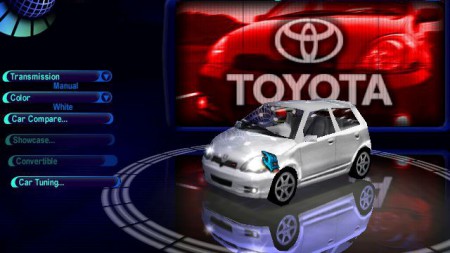The image shows a computer screenshot of a promotional page featuring a silver, compact Toyota van with four doors situated on a highly reflective, revolving platform. The platform, dark with a white circular edge, creates a perfect reflection of the car. Behind the van is the Toyota logo and the word "Toyota" in front of a red-tinted backdrop. To the left of the image, a side menu appears on the webpage with light blue text on a dark blue background, listing buttons like transmission, color, car compare, showcase, convertibles, and car tuning. The entire setup, indicating a showroom-style presentation, emphasizes the vehicle's features and is designed for viewing or comparing cars online.